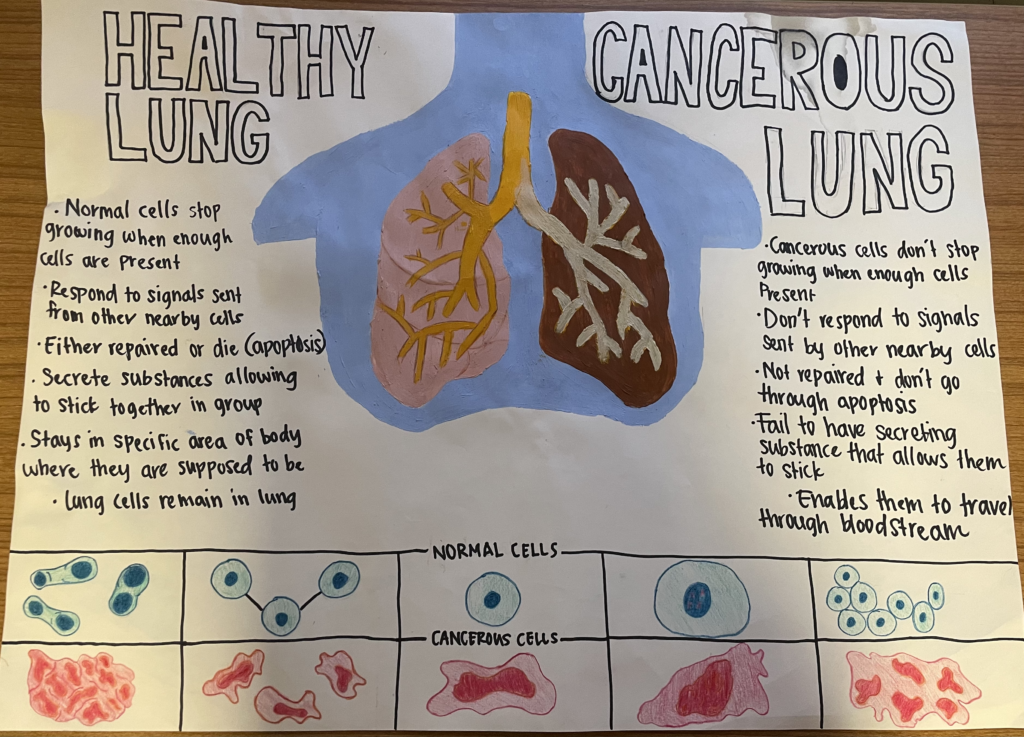This image is a detailed educational poster likely created by a high school or university student as part of a presentation. The poster compares a healthy lung to a cancerous lung and is displayed on a white poster board. At the top, the title "Healthy Lung" is on the left and "Cancerous Lung" is on the right.

The left section, under "Healthy Lung," explains that normal lung cells:
- Stop growing when enough cells are present.
- Respond to signals from nearby cells.
- Either repair or undergo apoptosis (programmed cell death).
- Secrete substances that allow them to stick together and remain in their specific area within the lung.

Below this, there is an illustration of a healthy lung, depicted in pink with yellow bronchi and bronchioles running through it.

The right section, under "Cancerous Lung," contrasts this by explaining that cancerous lung cells:
- Do not stop growing when enough cells are present.
- Do not respond to signals from nearby cells.
- Do not repair themselves or undergo apoptosis.
- Lack the substances needed to stick together, which enables them to travel through the bloodstream.

The accompanying illustration of a cancerous lung shows a brown lung with white or cream-colored bronchi and bronchioles.

At the bottom of the poster, a grid comparison between normal and cancerous cells is shown. The normal cells are pictured in five blue-toned boxes, while the cancerous cells are depicted in five red-toned, blobby-shaped boxes. This visual aid emphasizes the structural differences between healthy and cancerous cells.